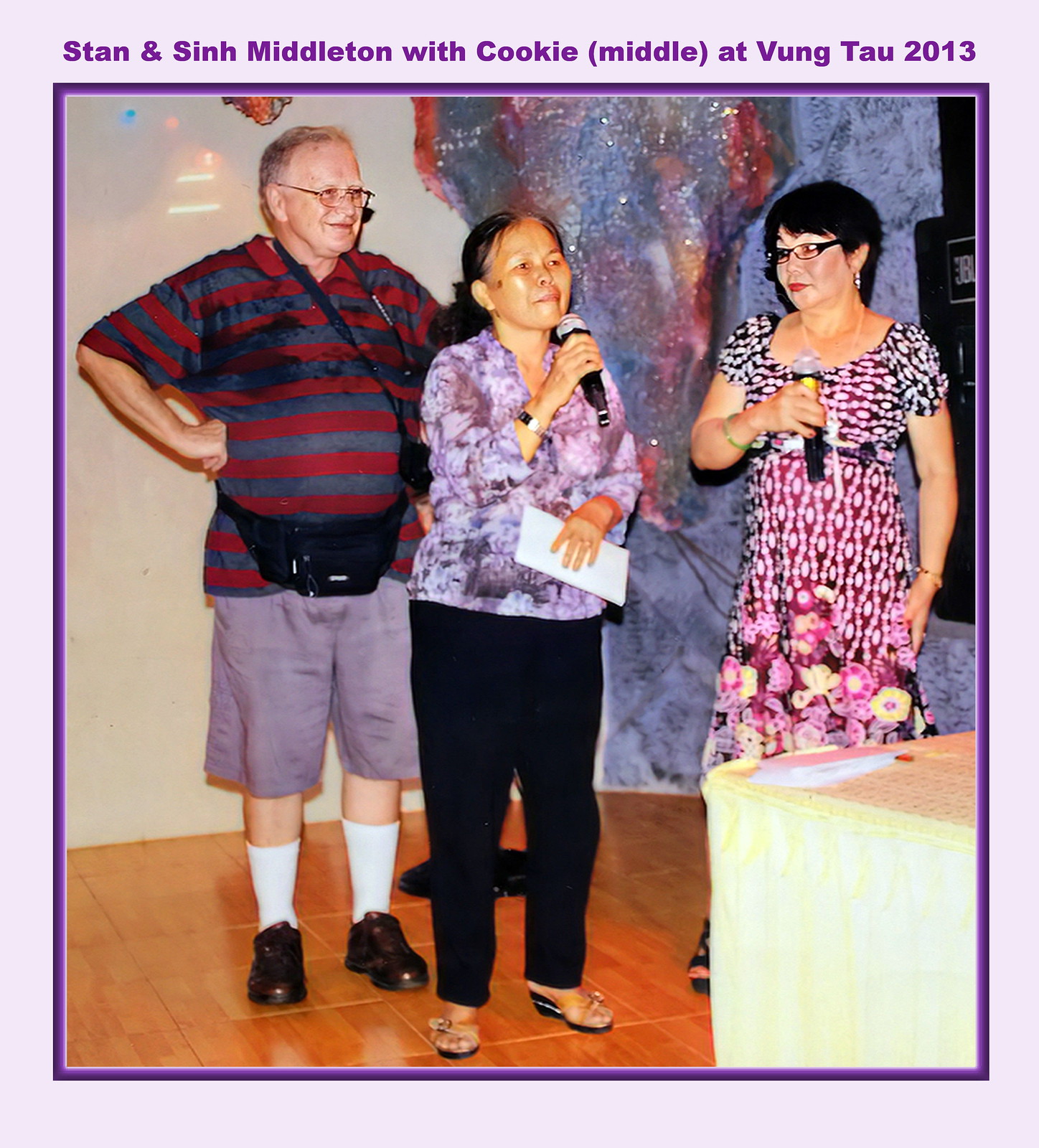The image displays an indoor setting with three people. In the center, a woman with tanned skin, dark brown hair tied back, and glasses is holding a microphone in her right hand and a white piece of paper in her left. She is dressed in a purple floral top and black trousers. To her left stands a man wearing a red and blue vertical striped top, a bum bag around his waist, light blue shorts, long white socks, and black shoes. To her right, another woman with short brown hair, glasses, and red lipstick is also holding a microphone. She wears a printed floral dress. The flooring is an orange wooden color, and the background features a white section on the left and a shimmery purple section on the right. The border of the photo is light purple with dark purple text reading "Stan and Sin Middleton with Cookie in the middle at Vung Tau 2013."